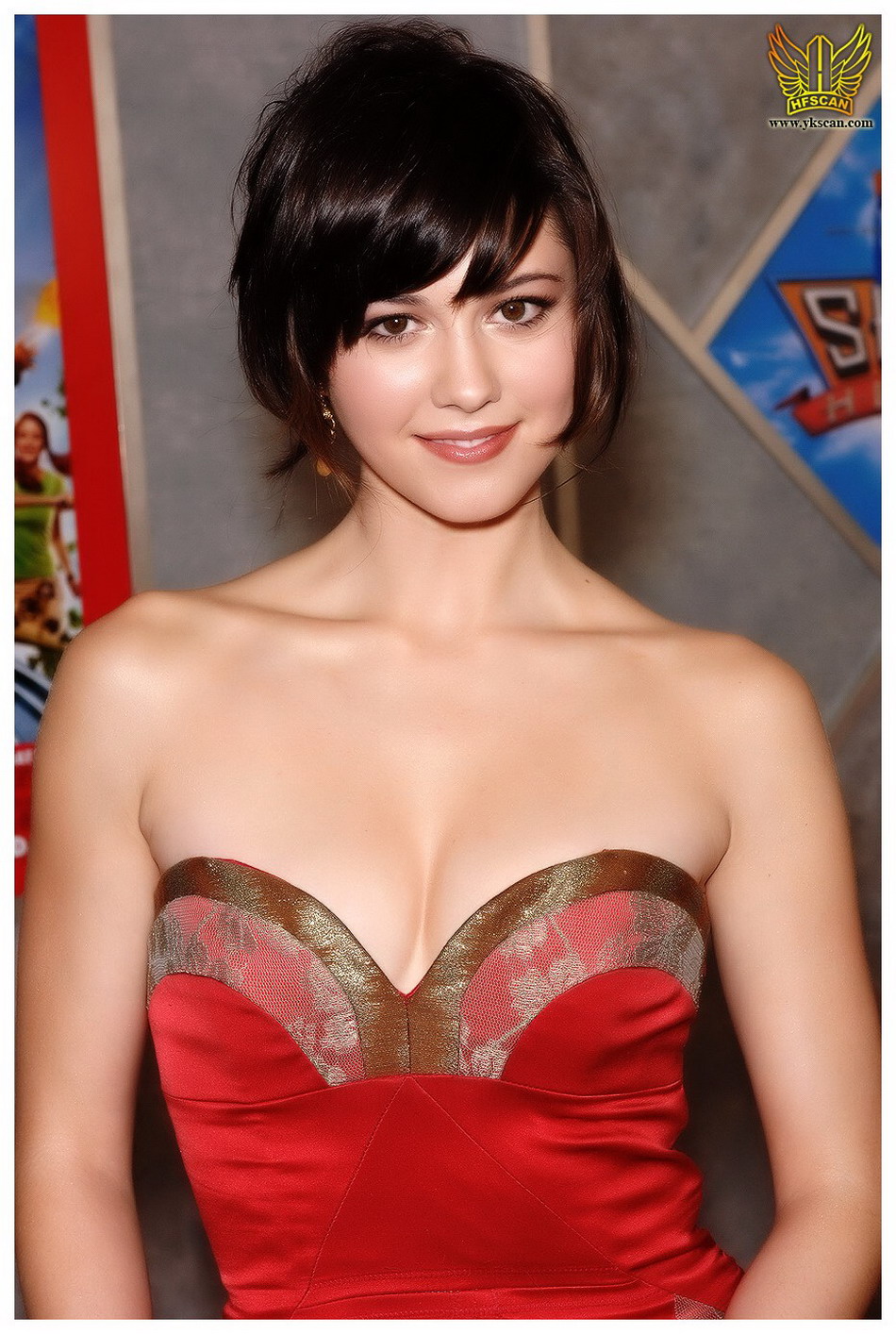This is a detailed photograph of a young woman, possibly a teenager or in her 20s, posing in a vibrant red dress with a low neckline. She is smiling warmly at the camera, her black bob-cut hair framing her face. Her arms rest casually at her sides, and she stands confidently with her shoulders squared. The backdrop suggests a formal event, perhaps a movie premiere, with an array of sponsor logos and slogans, evoking the feel of a red carpet setting. Notably, in the upper right-hand corner of the image, the text "HF Scan" along with the website "ykscan.com" are visible. The backdrop features colors including royal blue, orange, light red, and gray, enhancing the glamorous atmosphere. The lighting highlights her shoulders and cheeks, indicating that the photo was taken indoors, though it is unclear if it was captured during the day or night. The setting, her poised stance, and the professional backdrop hint that she might be a young actress who looks vaguely familiar.